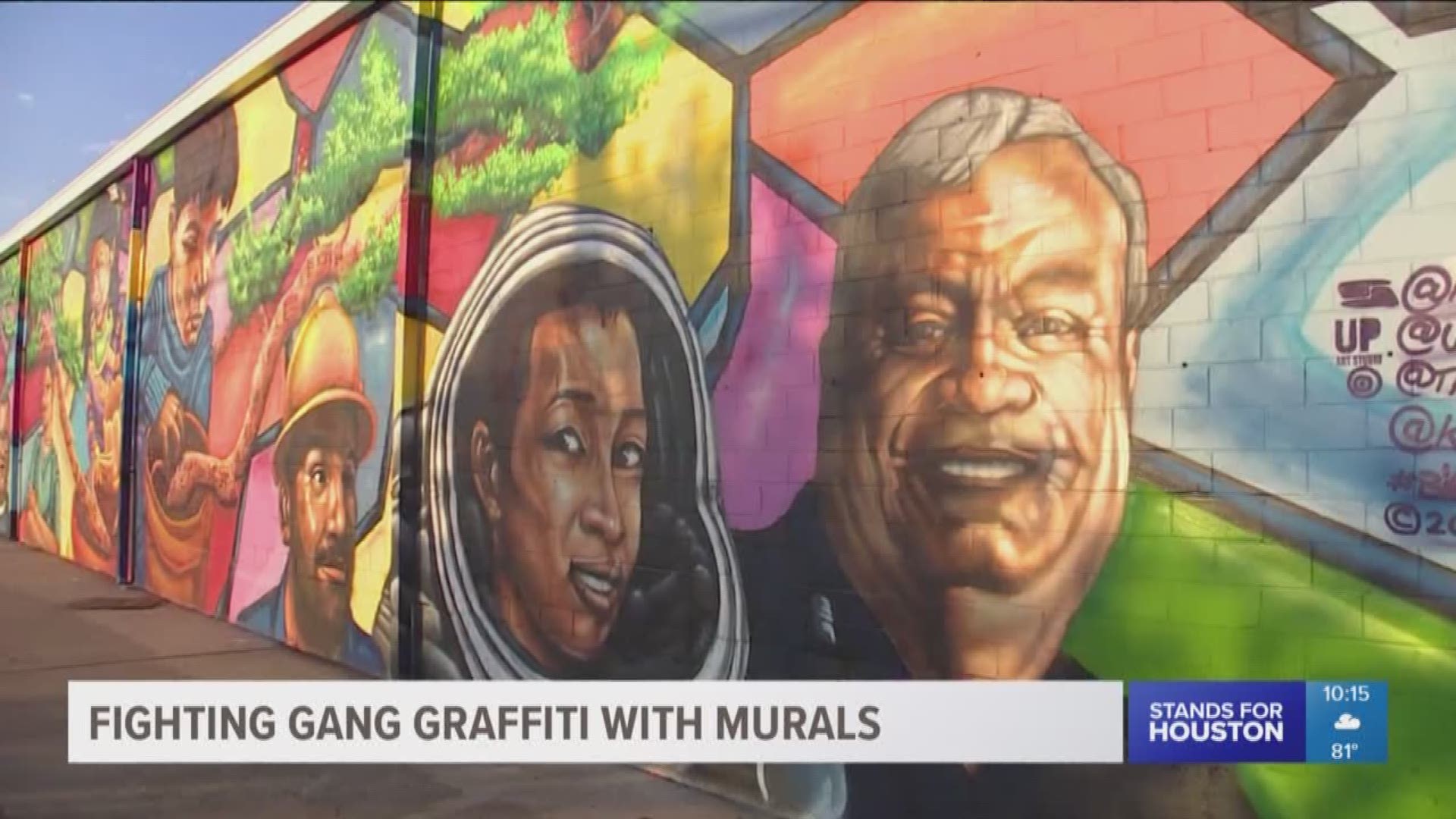The image features a large brick wall adorned with an extensive and intricately detailed mural. The mural, viewed at a diagonal angle, spreads from a wider section on the right to a narrower part on the left. Dominating the bottom section, a white rectangular banner prominently displays the bold, black capital letters: "FIGHTING GANG GRAFFITI WITH MURALS." Adjacent to this banner, on the right, a small blue rectangle with white text reads "STANDS FOR HOUSTON." Further right, a light blue square portrays a simplified weather report, showing "1015" at the top, a white cloud icon, and "81 DEGREES" beneath the cloud.

The mural itself is vibrant and realistic, featuring numerous portraits interspersed with geometric shapes and colorful backgrounds. Among the figures is an older man, perhaps in his 60s, with a smiling face devoid of facial hair, and a woman in what appears to be an astronaut suit, her face visible through the helmet's visor. The mural seamlessly merges various elements, including trees and other figures, creating a rich tapestry of artwork. On the right-hand side, some text is visible, likely the artists' signatures, although it's too small to decipher. The setting also includes glimpses of a gray sidewalk at the bottom left and a blue sky in the upper left corner.